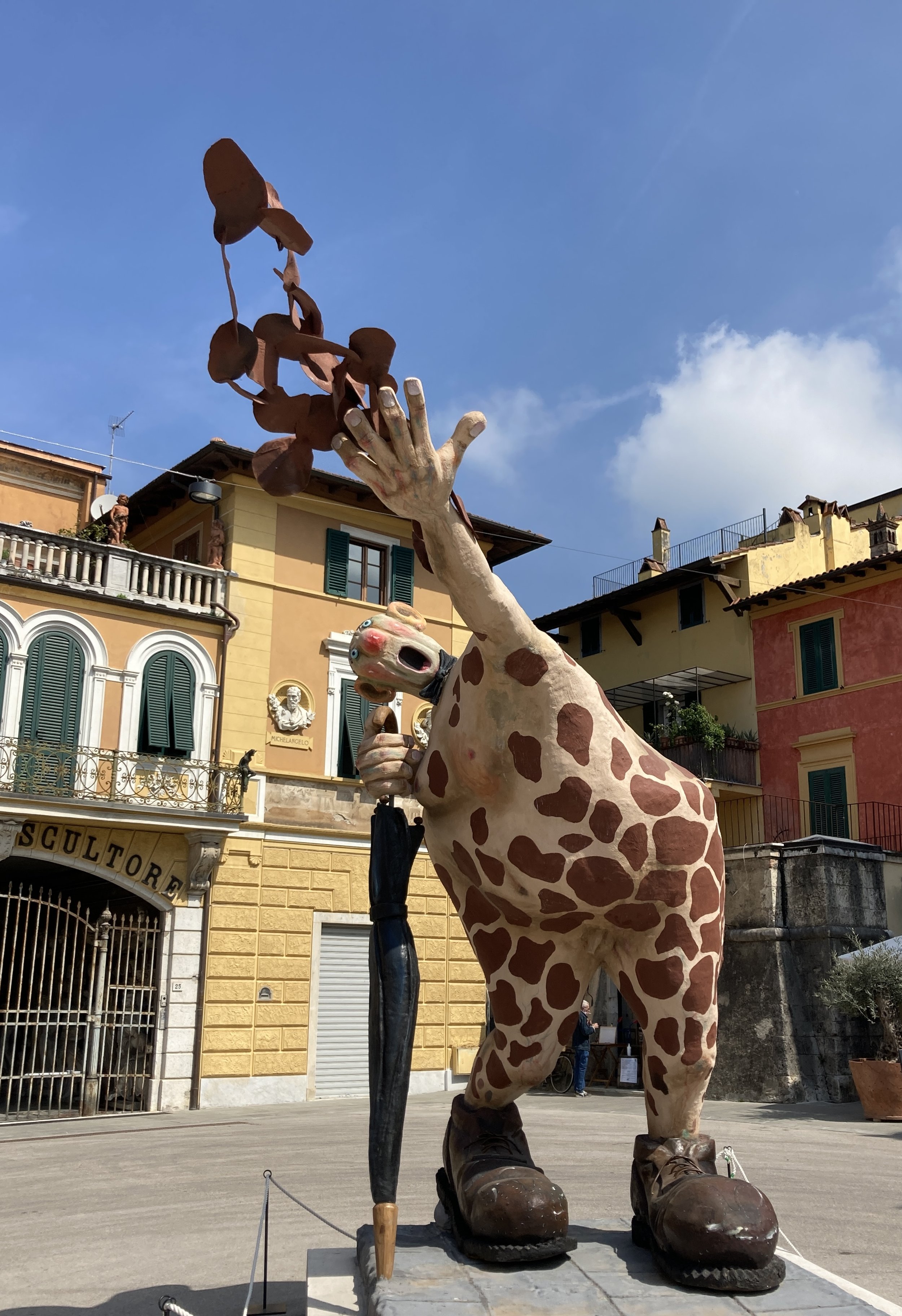In this vibrant daytime photograph, a whimsical statue depicting a half-man, half-giraffe figure stands prominently on a sunny sidewalk beneath a clear blue sky. The statue features the face of a man with wide, surprised eyes and an open mouth, atop a body that widens toward the bottom with a giraffe pattern. One arm is extended upward, appearing to toss or catch objects, while the other holds an umbrella. The statue is adorned with large brown boots, adding to its eccentric charm.

Behind the statue, several colorful buildings populate the scene, including a yellow building with a middle balcony and white arched windows with green panes and curtains. This yellow building bears the sign "Scultore" above a white gate. To the right of this structure, a pink (or possibly red) building and another yellow building can be seen. The asphalt below gleams under the sunlight, adding to the overall cheerful atmosphere of the setting, which is reminiscent of an amusement park or a creatively designed urban space.